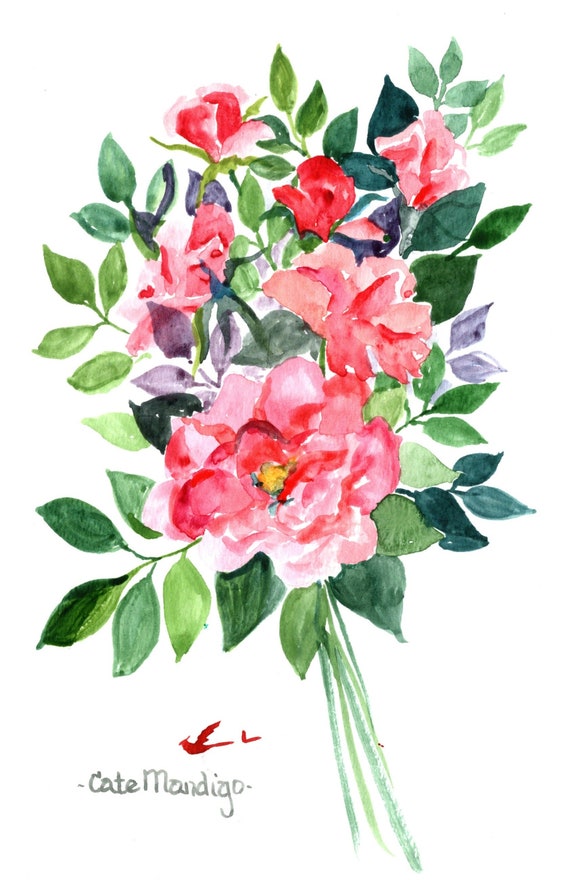This image is a delicate illustration, likely created with pen and ink or watercolor, featuring a bouquet of flowers against a completely white background. Emerging from the bottom are several green stems that support an array of leaves, which range from dark green to a lighter blue-green, with some additional purple hues scattered throughout. Encircling the bouquet are seven flowers in vibrant shades of pink, dark pink, red, and white, each with a striking yellow spot at the center, suggesting the pollen. Among the blossoms is a prominent, fully-bloomed rose, vividly detailed, while others are depicted as closed, stylized buds with an impressionistic style. In the bottom left corner, the artist's signature, "Kate Mandigo," spelled C-A-T-E M-A-N-D-I-G-O in gray ink, is accompanied by an image of two small red birds, adding a whimsical touch to the artwork.